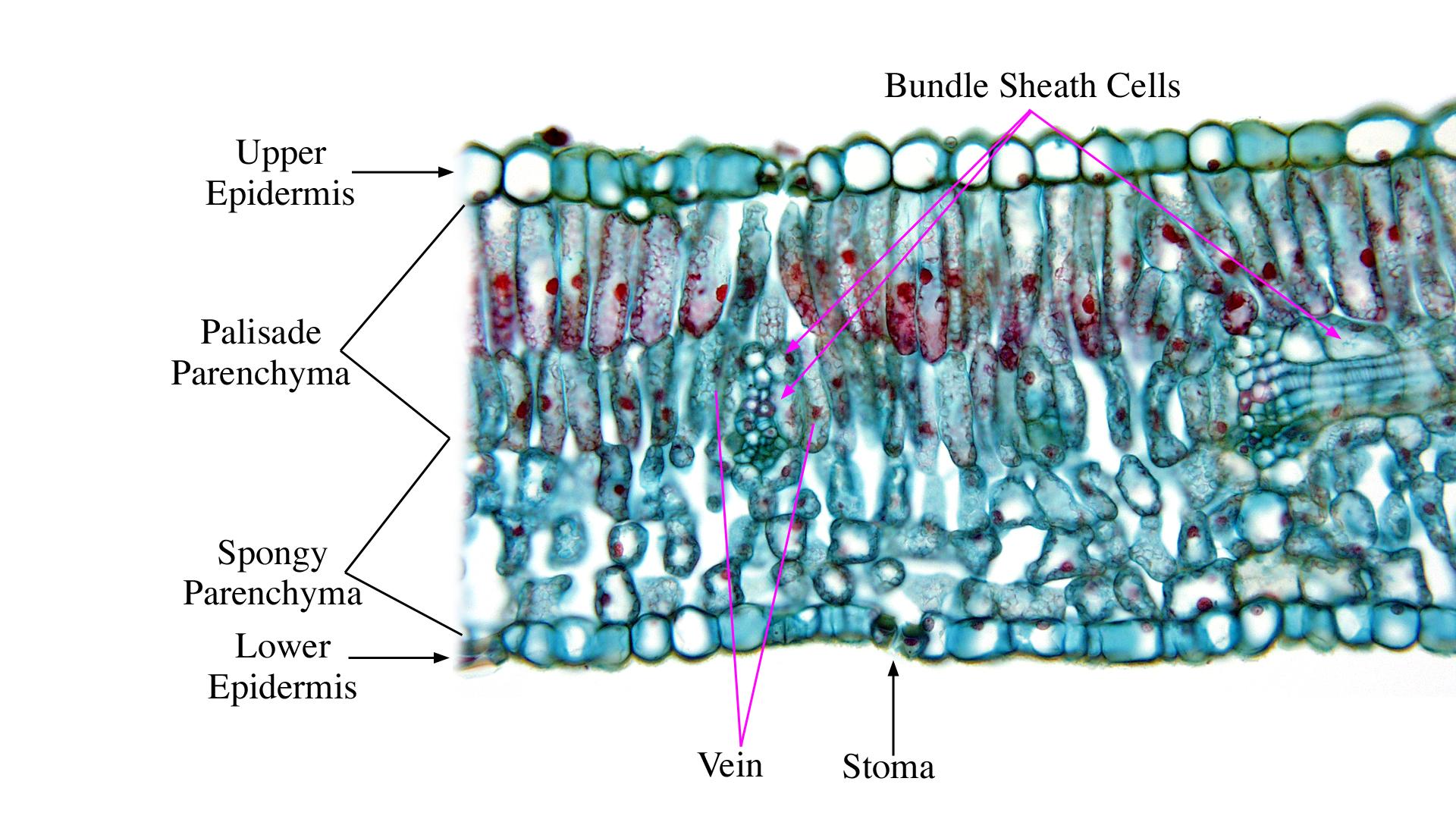The image depicts a detailed, labeled microscopic view of plant tissue, primarily highlighted in various shades of blue with red dots and streaks throughout. The composition showcases two distinct layers labeled as the upper epidermis and lower epidermis, both characterized by clusters of circular cells arranged horizontally across the top and bottom of the image. Between these layers, sections are identified as palisade parenchyma at multiple points, and spongy parenchyma is indicated with arrows pointing to several areas. Central to the image are the labeled bundle sheath cells, veins, and stomata. Overall, the image offers an intricate look at the cellular structure of plant tissue, with precise differentiation of its components.